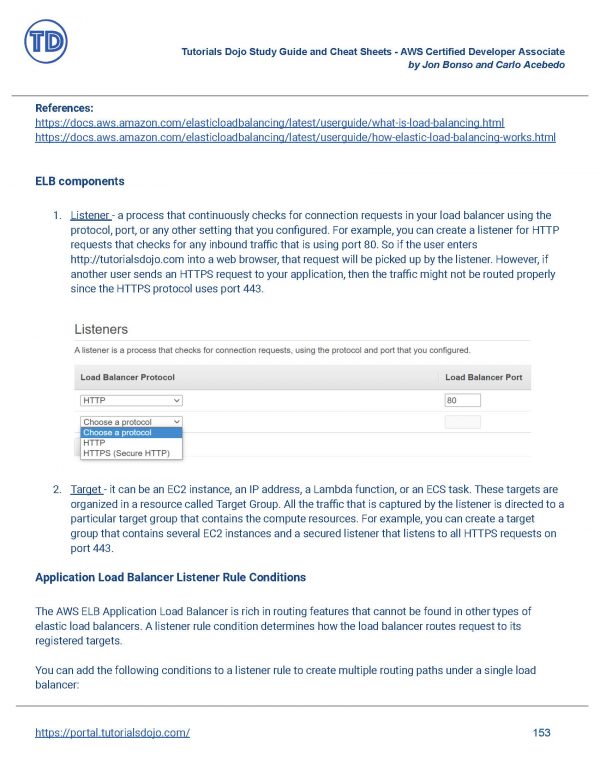This image showcases a page from a tutorial. In the upper left corner, there is a circular company logo outlined in dark blue, featuring the capital letters "T" and "D" in dark blue, with a white center. To the right, a dark blue title reads, "Tutorials Dojo Study Guide and Cheat Sheets – AWS Certified Developer Associate." Below this title, the authors' names are listed.

On the left side, a section titled "References" appears in bold dark blue font, followed by two URL links in dark blue. Below this, there is another bolded title, "ELB Components," indicating the beginning of a new section.

This section is numbered, starting with "1. Listeners," which is underlined with a dark blue horizontal line. Beneath this title, there is a description in dark gray text explaining the role of Listeners. There are two drop-down menus: the first, labeled "HTTP," has a white background, while the second is expanded to reveal selections. The first option, marked in dark blue with white text, reads "Choose a Protocol," followed by options "HTTP" and "HTTPS."

Further down, the text is labeled "2. Target," accompanied by a detailed description in dark blue writing. Another bolded subtitle reads "Application Load Balancer Listener Rule Conditions," providing further explanations below in dark blue text.